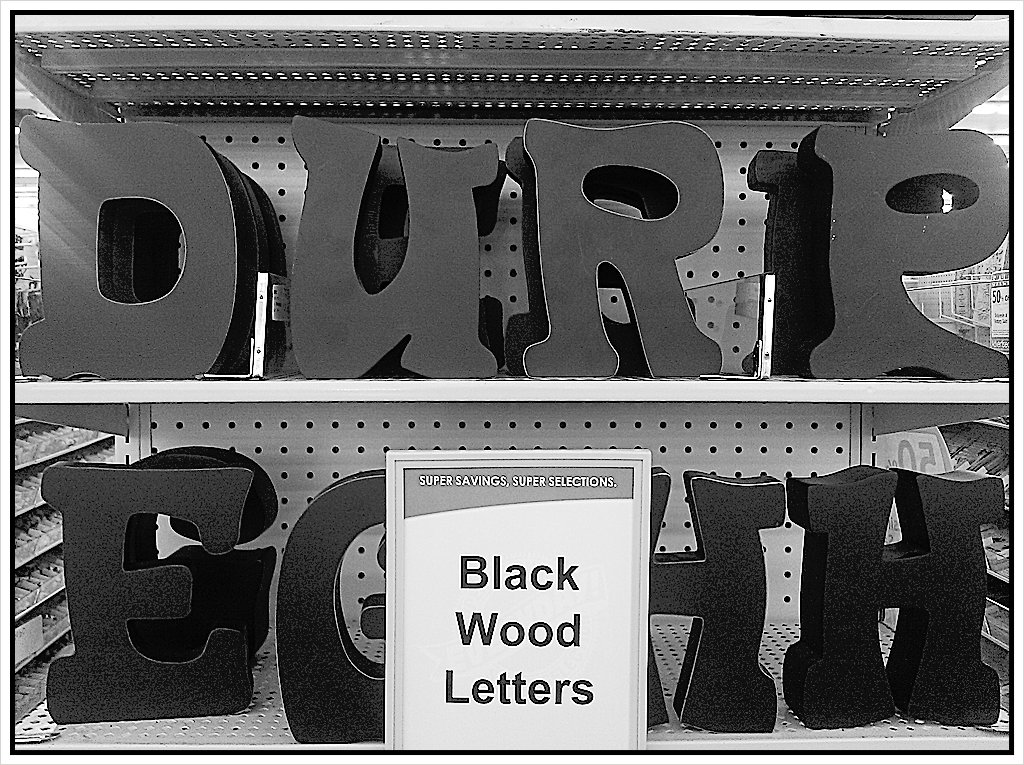A black and white photograph captures an organized display of wooden letters available for purchase in a store. The wooden letters are meticulously arranged on two shelves. At the center of the lower shelf, there is a prominent sign in a white frame that reads "Super Savings, Super Selections" above a white section with black font that labels the product as "Black Wood Letters." On the top shelf, the visible letters spell out "D-U-R-P." The lower shelf shows an incomplete sequence of letters "E-G-H-H," partially obscured by the sign. The photograph highlights the store's promotional efforts and the variety of wooden letters available for shoppers.